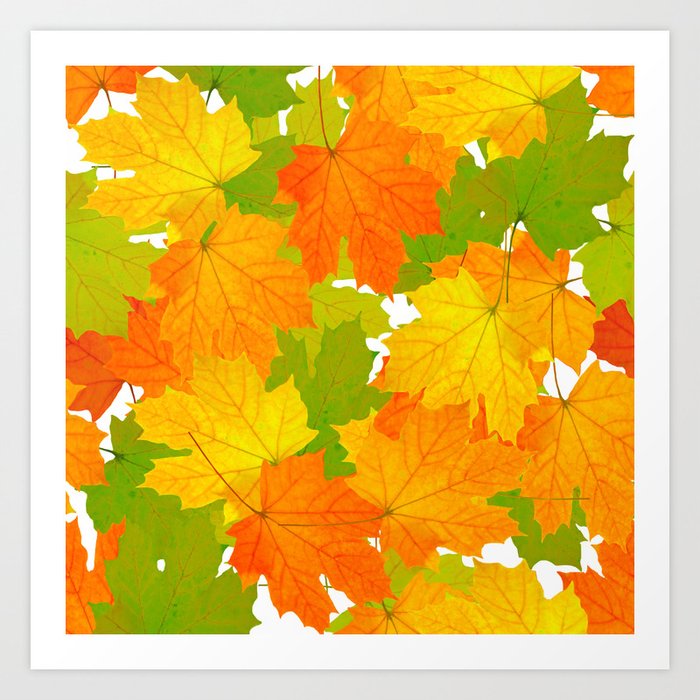The image is a detailed color photograph capturing a framed piece of autumn-themed art. This art piece is square in shape and features an off-white frame complemented by a white matting. The main canvas showcases a collection of multicolored leaves—primarily maple leaves—spanning various shades of orange, yellow, green, and even a distinct red one. The leaves lie flat, overlapping each other, against a stark white background, creating the impression of having been randomly scattered by the wind. The overall composition emphasizes the colors and textures of autumn foliage, providing a flat, top-down view. The artwork is hanging against an off-white or beige wall.